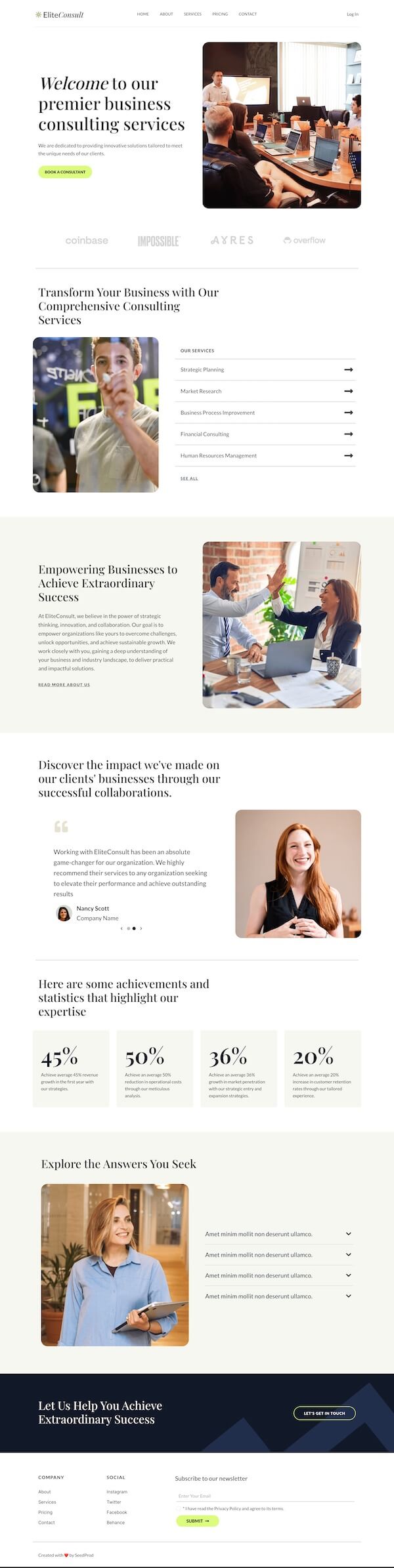The image is blurry, making the text difficult to read, but its general structure and elements are discernible. At the top, there is a headline or title. Below the title, on the left side, more text can be seen, adjacent to a green line or button. To the right of this text, there's a picture, possibly depicting a person and a table. Directly beneath this image are four words, which are unfortunately unreadable, followed by a couple of sentences.

Continuing downward, there's an image of a person above two columns of text. Below these columns, another picture appears with accompanying text: a line on the left side and a paragraph underneath. Below the paragraph, there are a few lines of text leading to another paragraph. Additionally, on the right side, there is a picture of a woman, with a few lines of text beneath it. 

Towards the bottom of the image, four gray boxes with text inside are present, followed by another picture of a woman wearing a blue shirt.